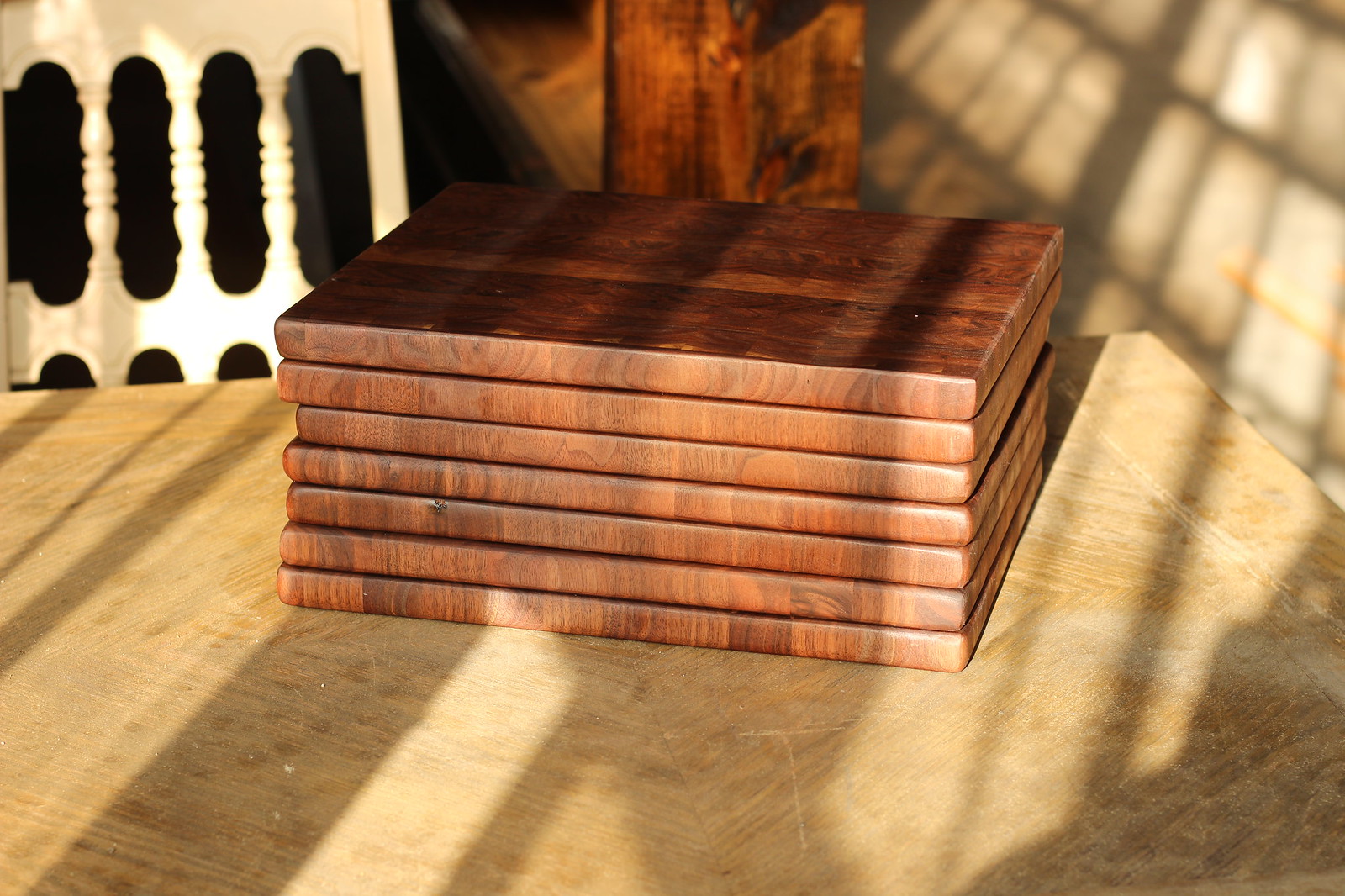The photograph, taken indoors, features a focal point of seven dark brown, rectangular wooden blocks or platforms stacked horizontally atop one another. These blocks rest on a light wooden table positioned centrally in the image. In the background on the left, there's a distinctive white chair with oblong holes in the backrest and spiral-shaped spindles between them. Further to the right of the chair, a piece of dark wooden furniture is visible. The wooden blocks, all equal in size, exhibit intricate, darker brown designs. Light and shadows interplay across the table and the blocks, adding to the textural richness of the scene.